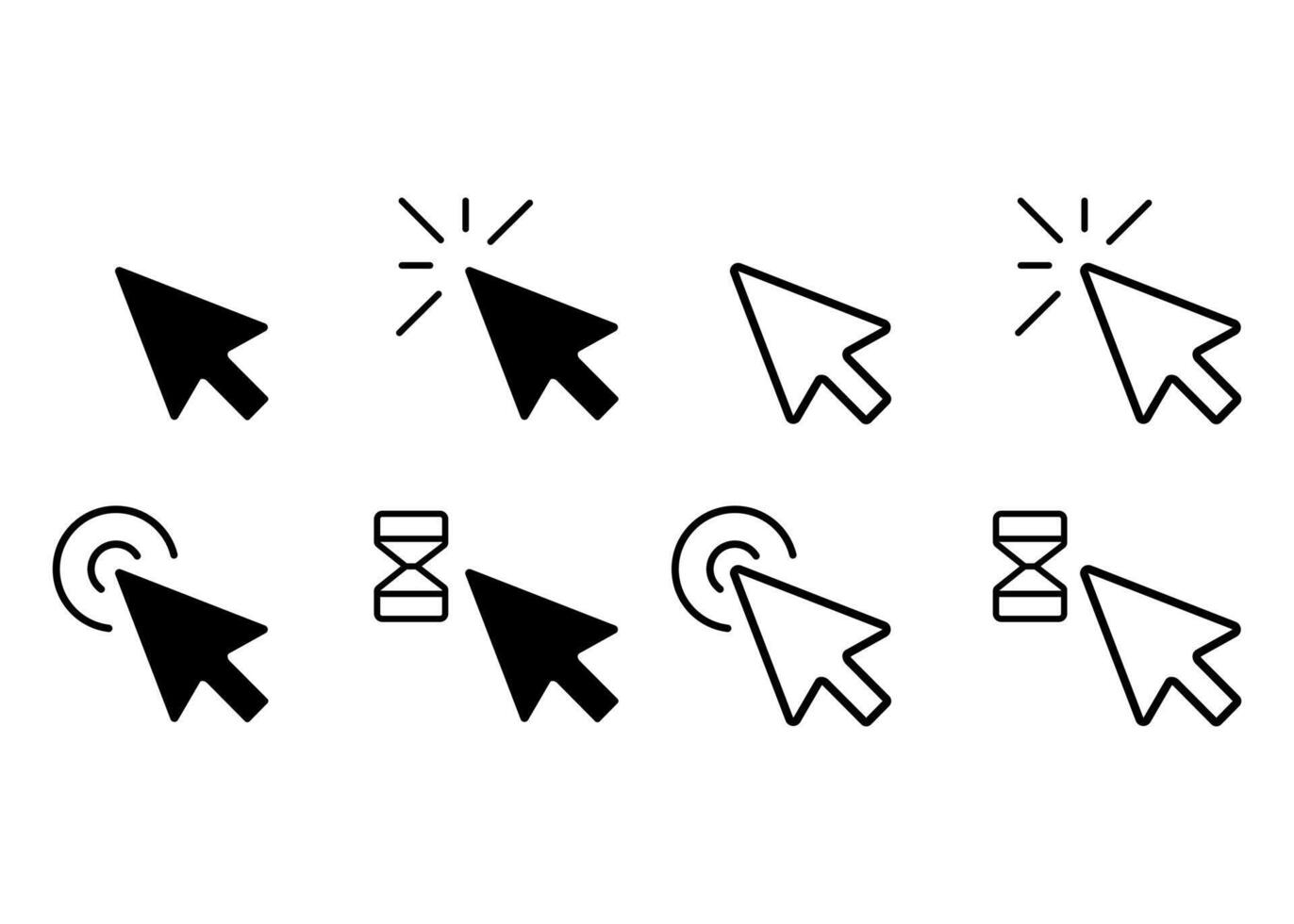The image features a grid of eight arrow cursors set against a stark white background, arranged in two rows of four. The top row starts with a black cursor arrow followed by another black arrow featuring some hand-drawn lines, then a white arrow with a black outline, and finishes with a similar white arrow also adorned with hand-drawn lines. The bottom row mirrors this pattern with some variations: it starts with a black arrow, followed by another black arrow surrounded by C-shaped lines, then a black arrow next to an hourglass symbol, and ends with two white arrows, one with C-shaped lines and the other with an hourglass next to it. The arrow designs appear to be professionally rendered, yet the context of the image remains unclear. The uniform arrangement and minimalistic black-and-white color scheme enhance the sense of a controlled, possibly digital design.